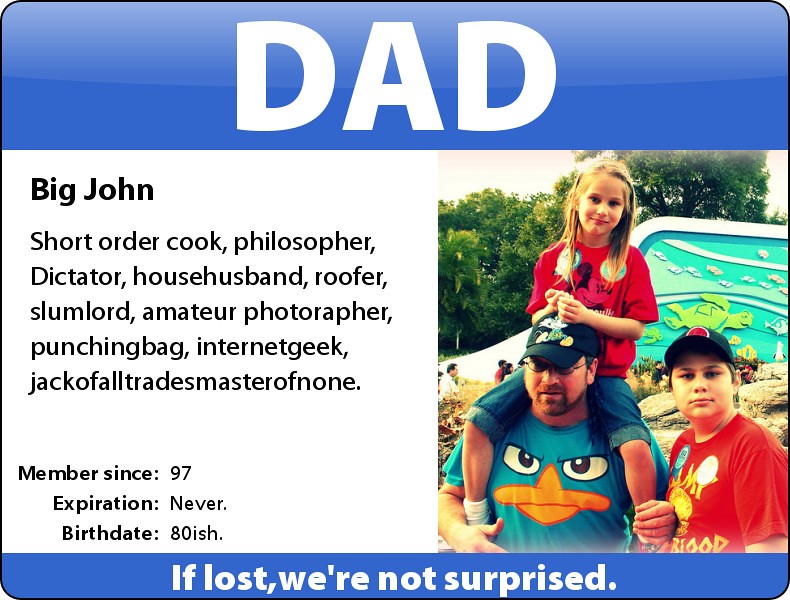The image depicts a whimsical, personalized membership card for "Big John," a multifaceted individual described as a short order cook, philosopher, dictator, house husband, roofer, slumlord, amateur photographer, punching bag, internet geek, jack-of-all-trades, and master of none. The card has a blue background with bold white letters spelling "Dad" at the top. It also reads "If lost, we're not surprised" in white text on the top strip.

The card features a photograph on the right side, showing a bearded man wearing round oval glasses, a black baseball cap, and a green Perry the Platypus t-shirt. He has a young boy with long blonde hair in a red Mickey Mouse shirt and blue shorts sitting on his shoulders. Next to him is an older teenager with short brown hair, holding a black baseball cap and wearing a red t-shirt. They appear to be a family enjoying an outing, likely at a park, with large rocks, trees, and what looks like a sea-themed mural with turtles and fish in the background.

Additional membership details include his status since 1997, with the card never expiring, and a birthday listed as "80-ish," implying a birth year in the 1980s. This Membership card humorously captures Big John's diverse and dynamic roles in life.